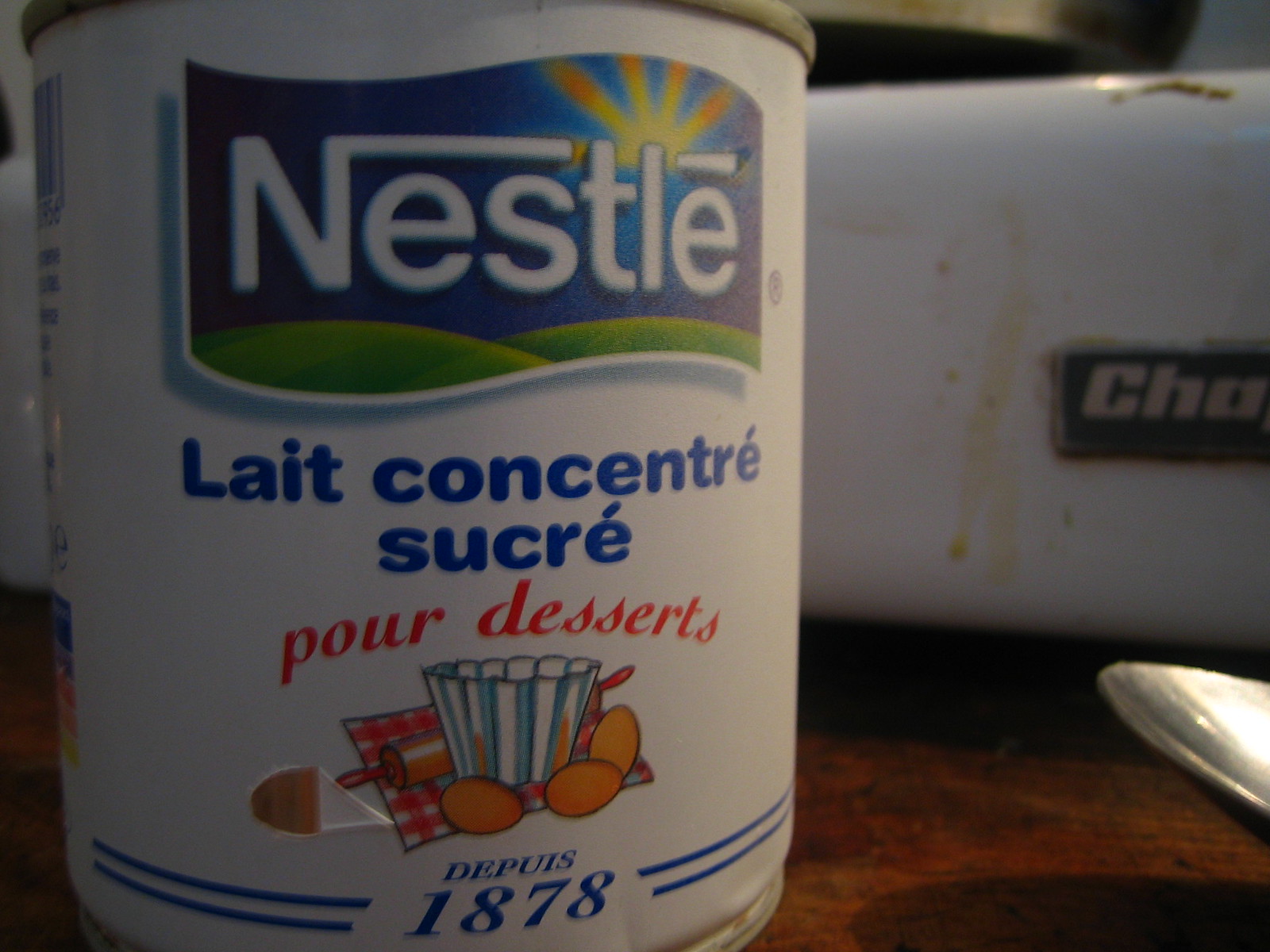The image showcases a vintage, close-up shot of a can of sweetened condensed milk. The can is primarily white, highlighting its aged and nostalgic appearance. Surrounding the top and bottom edges are thin metal rims, adding a subtle touch of industrial charm. The background is stark white, making the details on the can stand out prominently.

At the bottom of the can, a blue border consisting of two lines frames a segment of text. Inscribed within this border in blue font is the phrase "Dip Waste 1878," evoking a sense of historical significance. Just above this, there is an illustration featuring eggs, a mixing bowl, a rolling pin, and a red and white checkered towel, crafted to depict classic baking essentials.

Positioned above the illustration, in elegant red cursive, are the words "Poor Desserts," possibly alluding to a traditional range or product line. Above this text, written in blue font, is "Late Concentrate Sucre," which translates to condensed milk. Crowning the array of textual and illustrative elements is the iconic Nestle logo, signifying the renowned brand behind this timeless product. The combined elements conjure a sense of nostalgia and heritage, emphasizing the can's long-standing presence in culinary history.